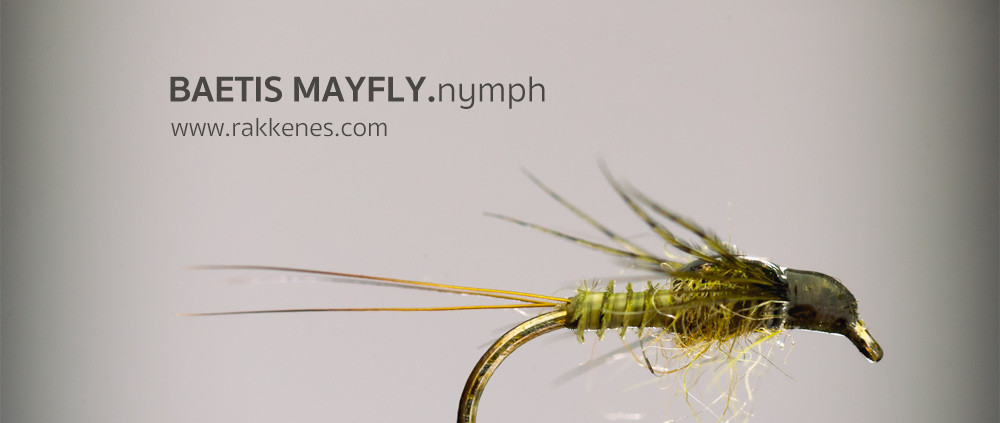The image depicts an advertisement for fly fishing bait, prominently featuring a highly detailed, artificial mayfly nymph. Positioned mainly on the right side but extending towards the left, this elaborate lure showcases an imitation insect with olive green coloring and intricate black-and-gold details on its beak-like face. The mayfly nymph is attached to a golden hook that curves gracefully towards the bottom of the image. The background is a gradient, transitioning from solid gray at the center to dark gray at the edges, adding depth and focus to the subject. In the upper left corner, the text "BAETISMAYFLY.NYMPH" is displayed in all caps, followed by the lowercase website "www.rakeens.com". The detailed craftsmanship of the bait, combined with the sharp, minimalist design of the advertisement, captures attention and appeals to fly fishing enthusiasts.